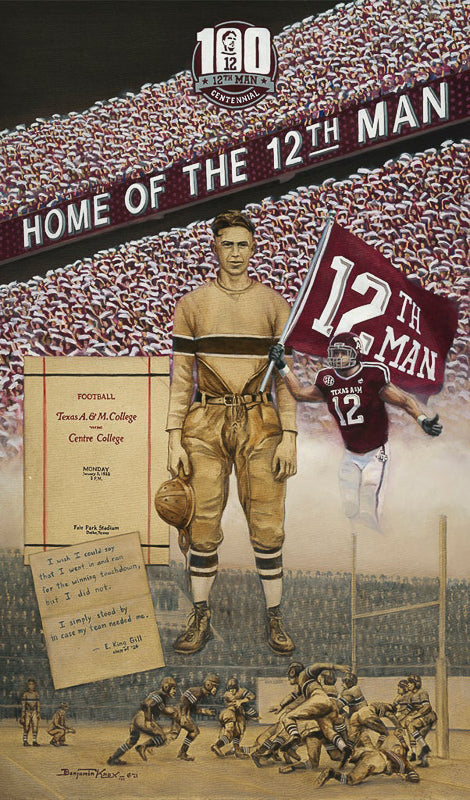This vertical rectangular poster prominently features a celebration of Texas A&M’s "Home of the Twelfth Man." Across the top of the poster, a diagonal dark purple strip spans from the lower left to the upper right, displaying the phrase "Home of the Twelfth Man" in bold white letters. Above this strip is a circular logo depicting "100," set against a background of a stadium packed with cheering fans.

Beneath the logo, the focal point includes two distinct football players, one in an old-time uniform and the other in a modern Texas A&M uniform. The man on the left is wearing vintage football attire, complete with old leather helmets, and is depicted holding his helmet. To his left, there's an old football program cover with the text: “Football, Texas A&M College versus Central College.” Below this program, a quote reads: "I wish I could say that I went and ran for the winning touchdown, but I did not. I simply stood by in case my team needed me. – E. King Gill."

To the right of the man in vintage gear stands another football player, donned in a contemporary Texas A&M uniform, holding a flag that proudly displays "12th Man" in white text. The modern player's jersey also features the number 12, reinforcing the 12th Man tradition. The overall design encapsulates the rich history and enduring spirit of Texas A&M's football culture, with a nod to the historical figure E. King Gill, the original 12th Man.